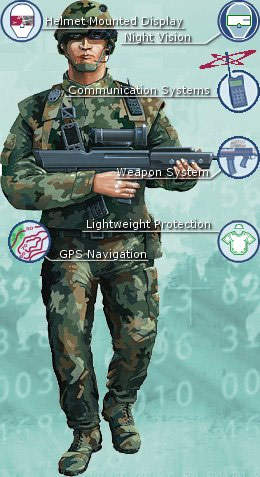The image depicts a detailed diagram of a soldier outfitted in full camouflage gear, including a helmet, while holding a black gun pointed to the right. The soldier's equipment is meticulously labeled with arrows and descriptions. At the top, there's a "helmet mounted display" featuring integrated night vision capabilities. The communication system includes a microphone extending to his mouth and a phone-like receiver on his left shoulder. His attire, comprised of traditional army green and tan camouflage fatigues, is described as "lightweight protection," likely indicating a flak jacket or bulletproof vest underneath. Additionally, "GPS navigation" is mentioned, although its precise location on the soldier is not detailed. The diagram, likely a computer-generated sketch, is set against a blue background that transitions from lighter blue at the top to a darker blue with white alphanumeric characters (0101362) in the lower half.